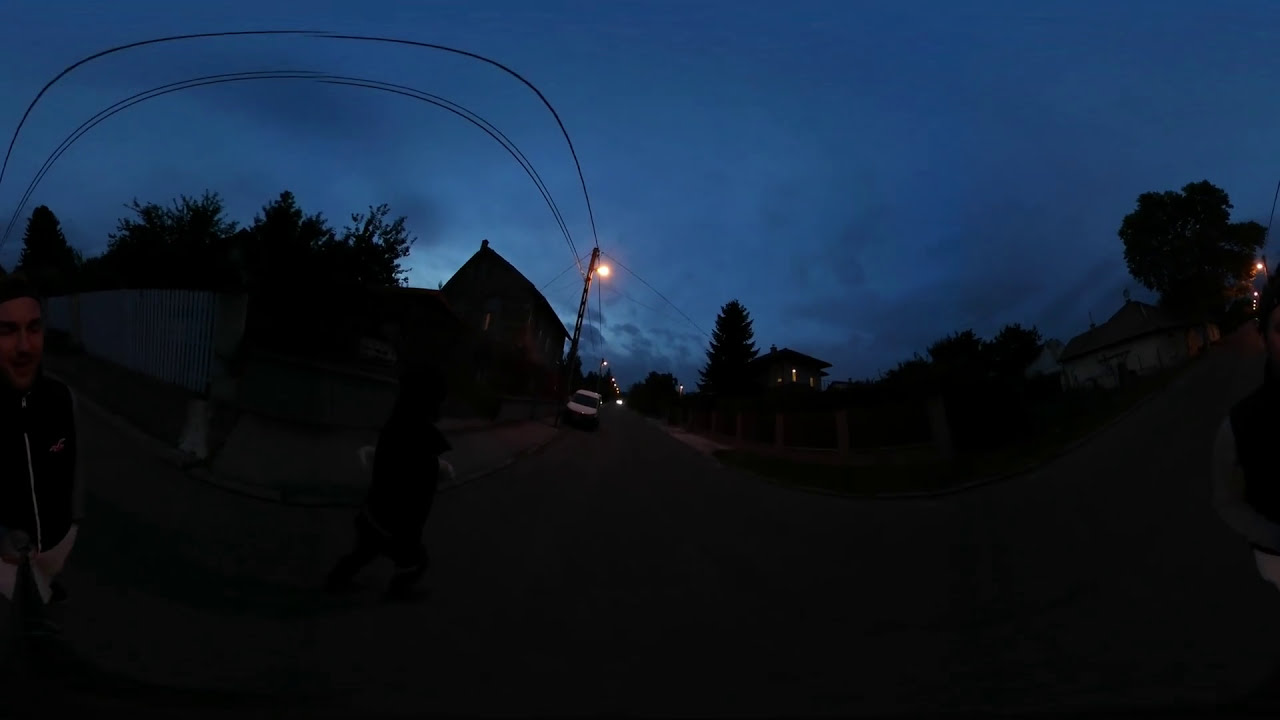The image showcases a nighttime outdoor residential setting with a clear dark blue sky, scattered gray clouds, and glimpses of moonlit areas despite the absence of the moon itself. Dominating the scene are the silhouettes of trees, houses, and rooftops, all mostly shrouded in darkness. A street lamp and several housing lights illuminate parts of the scene. A white fence runs along one side, beside which there are trees and a driveway with a white car partially inside a garage. Across the street, a white van is parked underneath another street lamp. The street and sidewalk are a muted gray, blending into the dim scenery. In the middle ground, two people are visible: one wearing a dark vest over a tan shirt and another in dark clothing with white accents, seemingly interacting with one another. In the forefront, a person in a black jacket stands with another figure nearby, who appears to be either standing or walking. The neighborhood feels quiet and calm, typical of an evening in a residential countryside.